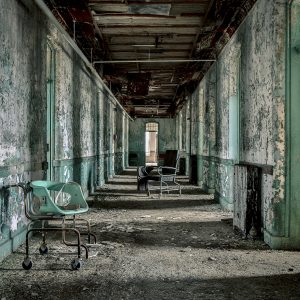This is an image depicting the interior of an abandoned building, possibly a former school or hall, located in Europe or a former European colony. The scene shows a dilapidated covered sidewalk with walls that appear to converge on a doorway at the end of the walkway. The structure is in a state of severe disrepair, with the floor completely destroyed and ceilings exposed, revealing wires and wooden planks. The walls are heavily weathered and peeling, with an accumulation of dirt and possibly mold. There is chipped paint, primarily exposing the underlying white and black with remnants of a mint green hue. Scattered across the middle of the walkway are various chairs, many of which have wheels. A teal or mint green wheeled chair is prominent in the foreground on the left side, while a darker chair, possibly gray or black, is situated further along the hallway. The sunlight can be seen streaming through open doors along the sides of this rundown passage, casting light on the tattered surroundings.